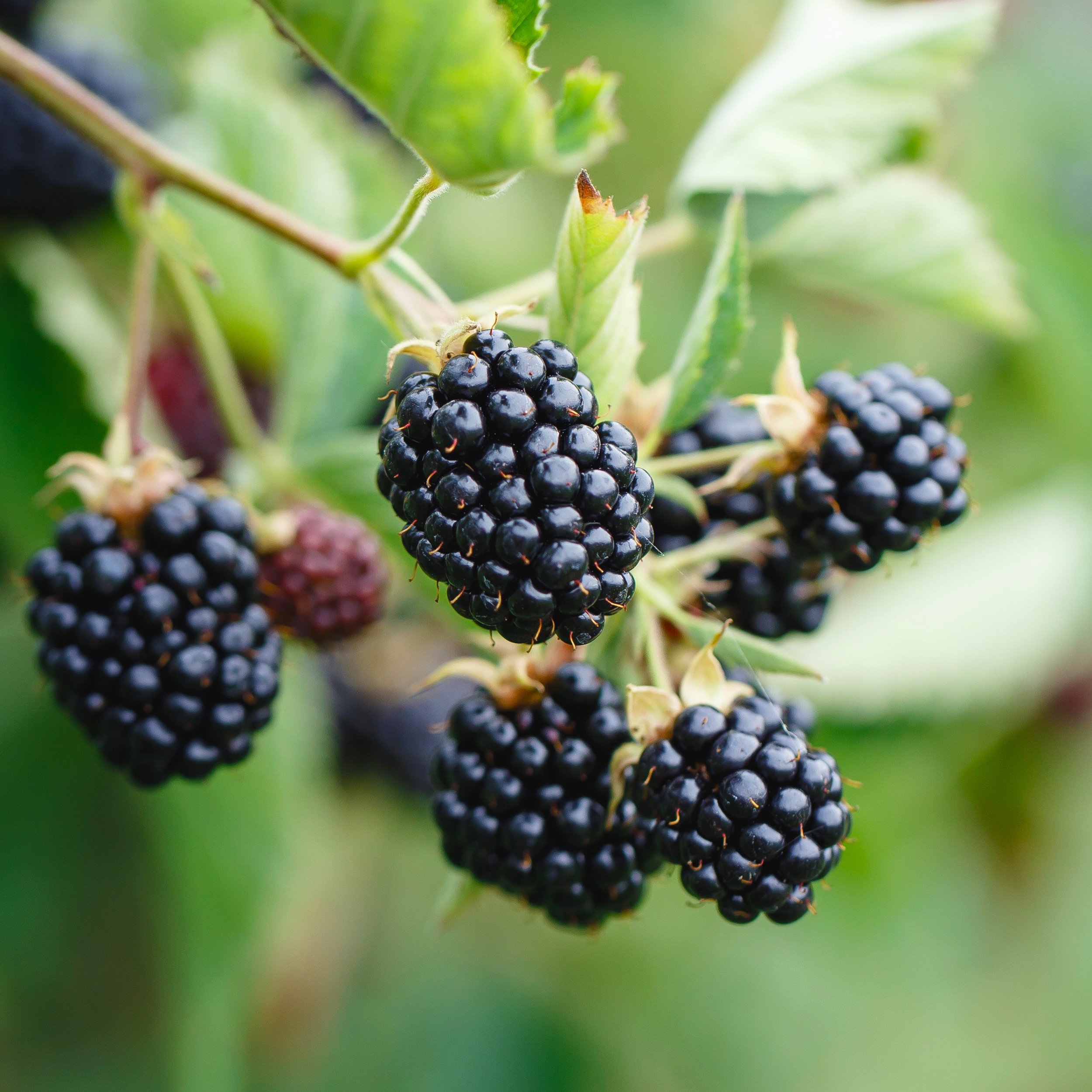This close-up, square image showcases a cluster of vibrant blackberries still attached to their vine. The foreground prominently features five or six fully ripened blackberries, exhibiting a deep purplish-black color with a shiny, plump appearance, indicative of their readiness for picking. These mature berries are clustered together on a greenish-brown stem that descends from the upper left corner of the photo. Surrounding the berries, the vine displays green leaves with slightly brown tips, and tiny light tan leaves are nestled right around the blackberry cluster. As the view extends into the background, the focus softens, revealing some less ripened blackberries in lighter shades of purple and brown. The backdrop remains largely blurry to accentuate the berries, suggesting a lush, leafy environment of green with hints of brown, likely from surrounding foliage. The image captures the intricate details of the mature blackberries, including the fine brown hairs on each drupelet, providing a vivid and intimate perspective on these wild, perfectly matured fruits.